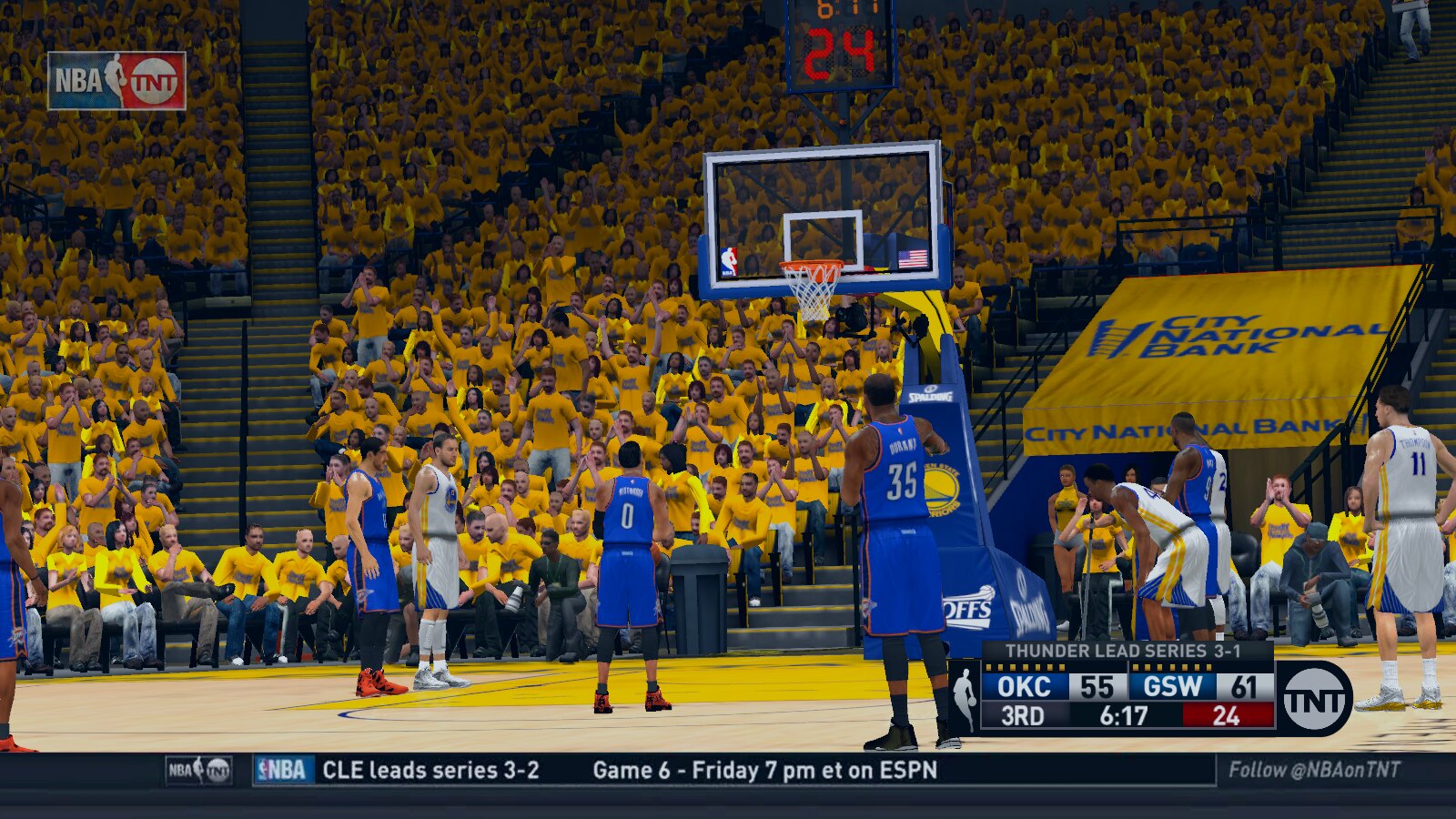The image captures the electrifying atmosphere of an NBA basketball game. A prominent NBA on TNT sign is visible among the enthusiastic crowd, highlighting the broadcast partnership. The court features players in contrasting uniforms: one team in blue with red trim and the other in white with blue and yellow accents. The scoreboard displays "NBA CLE lead series 3-2," indicating that the Cleveland team is ahead in the series, with Game 6 scheduled for Friday at 7 PM on ESPN.

Above the crowd, a large, eye-catching yellow banner with blue lettering reads "City National Bank," suggesting a significant sponsorship presence. The fans seated in this section are all wearing matching shirts, creating a sea of coordinated color that aligns with the banner's design. This visual unity indicates that many attendees likely received their tickets through the bank's promotional efforts, adding to the sense of community and excitement in the arena.